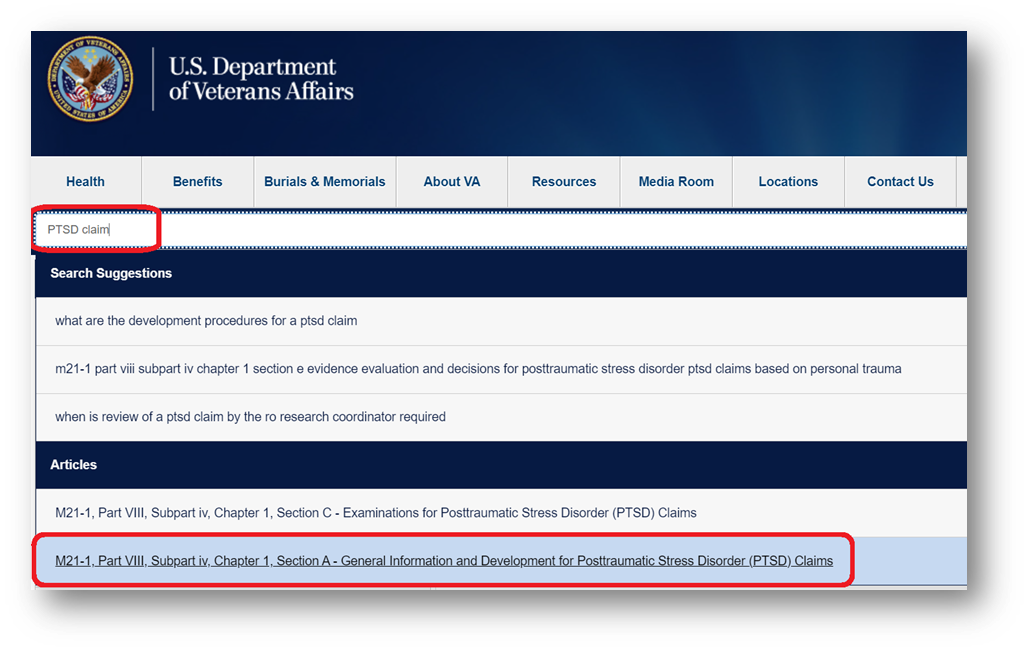This screenshot captures the homepage of the U.S. Department of Veterans Affairs website. The header of the site features a gradient background that transitions from a deep navy blue, almost black, on the left, to a lighter navy blue on the right. Positioned in the top-left corner is the circular emblem of the U.S. Department of Veterans Affairs, depicting an eagle and a flag, encircled by a gold ring. To the right of the emblem, separated by a short vertical white line, text appears in white that reads "U.S. Department of Veterans Affairs."

Beneath this header, the navigation bar stands out in white, presenting buttons for various sections of the website: Health, Benefits, Burials and Memorials, About VA, Resources, Media Room, Locations, and Contact Us.

Prominently featured in the centre of the screen is a red-highlighted search bar with the query "PTSD claim" entered. Below the search bar, a dark navy strip displays in white text, "Search suggestions," followed by detailed search results: 

1. "What are the development procedures for a PTSD claim? M21-1, Part VI, Subpart iv, Chapter 1, Section E, Evidence Evaluation and Decisions for Post-Traumatic Stress Disorder (PTSD) Claims Based on Personal Trauma"
2. "When is review of a PTSD claim by the RO research coordinator required?"

Further down, another navy bar with white text reads "Articles," followed by links to various articles and sections:
- "M21-1, Part VI, Subpart iv, Chapter 1, Section C, Examinations for Post-Traumatic Stress Disorder (PTSD) Claims."
- A highlighted link, encircled in red, points to "M21-1, Part VI, Subpart iv, Chapter 1, Section A, General Information and Development for Post-Traumatic Stress Disorder (PTSD) Claims."

This detailed depiction offers users a clear and structured insight into navigating PTSD-related information on the VA's website.